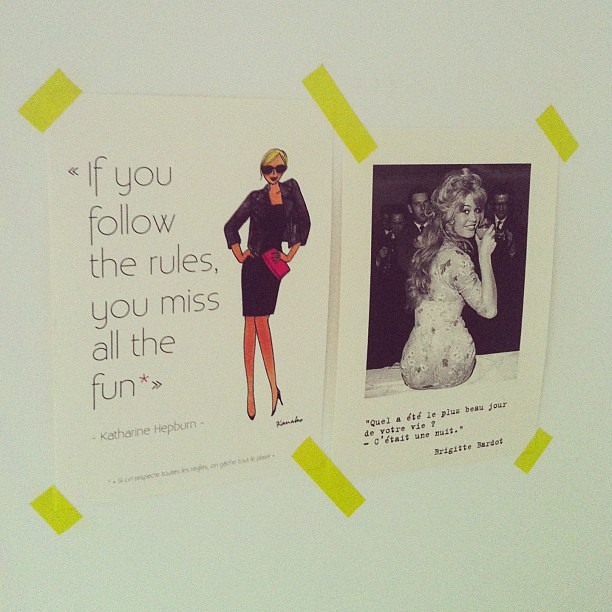This detailed image features two photos affixed to a white wall using bright yellow tape. The first photo on the left showcases a blonde woman in a black dress, blazer, and high heels, accessorized with a red (or pink) pocketbook and black sunglasses. She stands confidently with her hands on her waist and one leg tilted inward. This image is paired with a quote by Katherine Hepburn that reads, "If you follow the rules, you miss all the fun."

To the right, the second photo captures a lively party scene. A woman with long curly hair and her back turned to the camera is looking over her shoulder while holding a drink to her mouth. Behind her, a couple of men in suits are visible. At the bottom of this photo, a French quote is inscribed, attributed to Brigitte Bardot.

Both women in the photos are white, and the vibrant yellow tape draws attention to these vintage, fashionable snapshots on the wall.